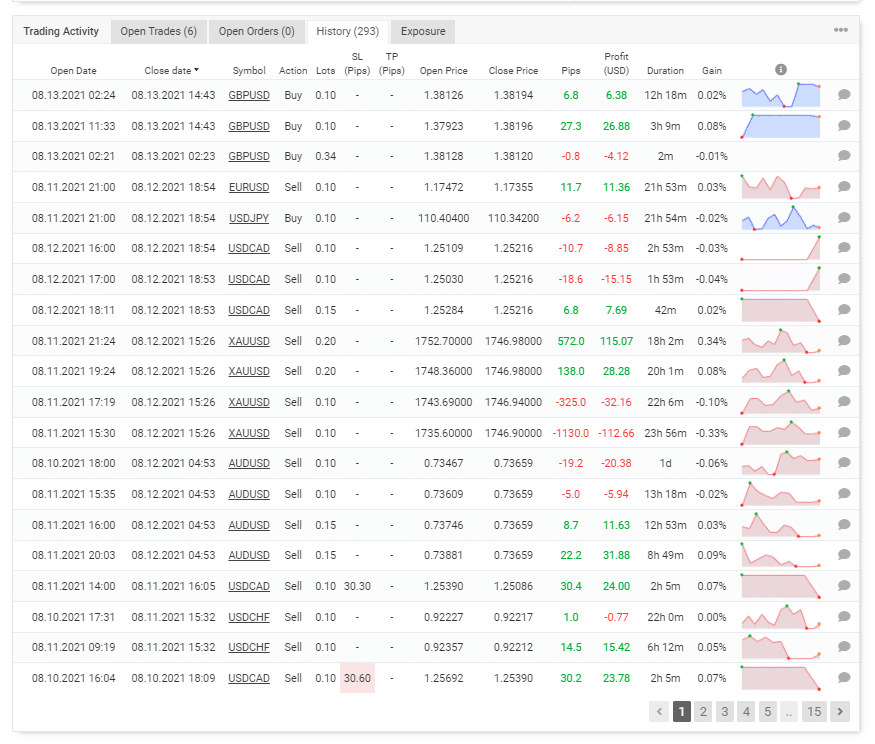A detailed caption for the image in question:

The image is a cropped screenshot of a trading activity panel from a stock trading website. The interface features a grey header with multiple tabs for navigation: "Trading Activity," "Open Trades," "Open Orders," "History," and "Exposure." In the upper right corner of the header, there is an ellipses icon for additional options or settings.

The "History" tab is currently selected, which is indicated by a (293) in parentheses next to it, suggesting this number of historical trades. Directly below the grey header, a comprehensive table is organized with vertical categories across the top: "Open Date," "Closed Date," "Symbol," "Action," "Lots," "SL" (Stop Loss), "TP" (Take Profit), "Open Price," "Closed Price," "Pips," "Profit," "Duration," "Gain," and an eye icon. To the right side of the panel, there are graphs aligned vertically alongside a chat bubble icon.

Entries under the "History" tab are listed sequentially. The top entry shows an open date of August 13, 2021, at 2:24, and a closed date of August 13, 2021, at 14:43. The detailed history continues down the page, which is labeled as page 1 of the history. At the bottom right corner, page navigation controls are visible, allowing users to go back or forward through the history using arrows or by clicking on specific page numbers.